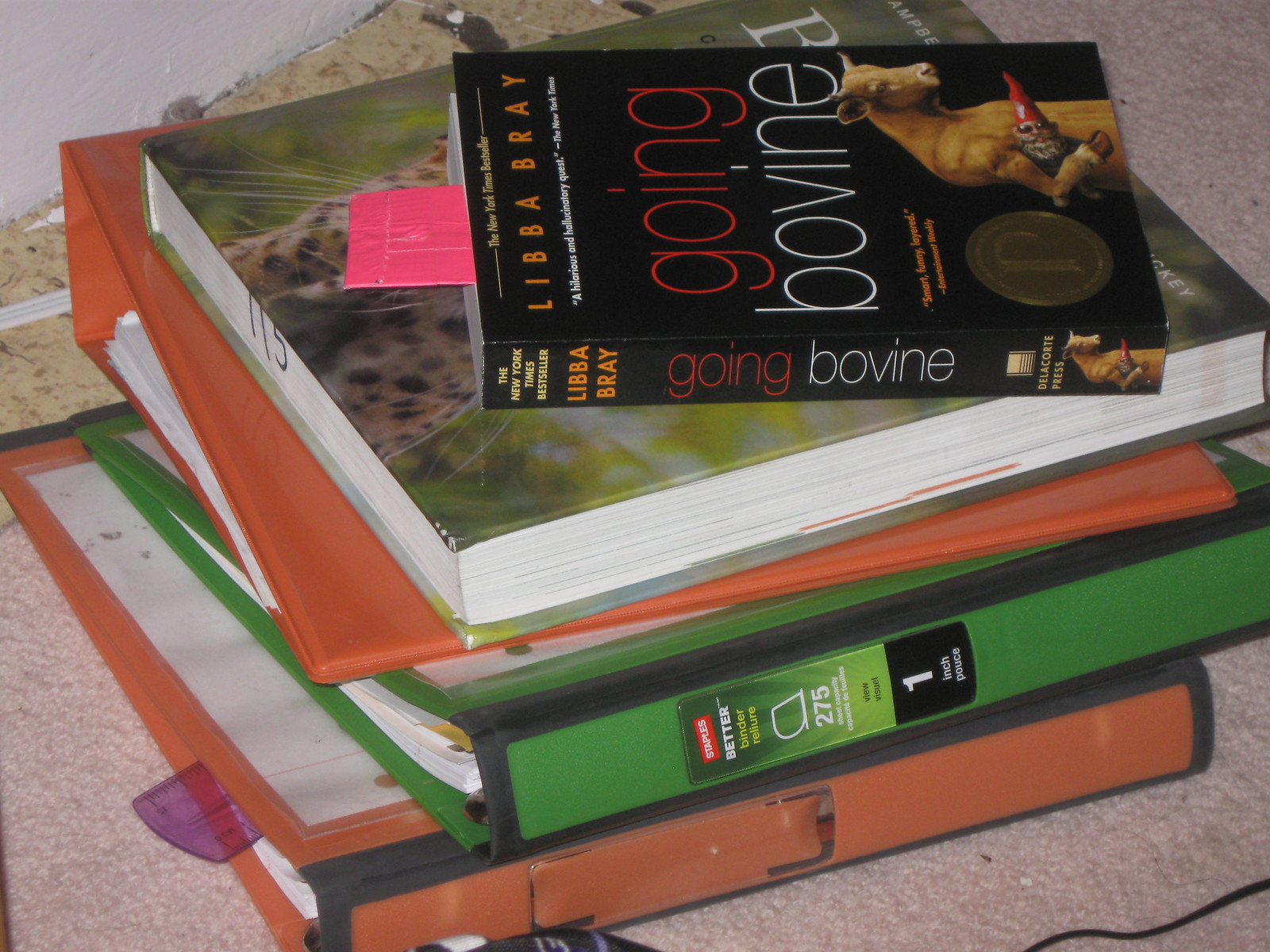This photograph features a neatly stacked pile of books and binders on a light grayish floor. The composition is more landscape-oriented, offering a close-up view of the items. On top of the stack is a black paperback book titled "Going Bovine" by Libba Bray, featuring a whimsical cover image of an upright cow holding a garden gnome. The spine, marked with "New York Times bestseller," matches the title and author's details, and a circular gold medal indicating an award is imprinted in the lower left corner of the cover. A neon pinkish-red bookmark peeks out from the middle of this book.

Beneath the paperback is a thick textbook, mostly green with hints of a cheetah illustration on its partly exposed cover. Following the textbook are three differently colored binders. At the bottom lies an orange binder with a purple translucent ruler sticking out, a white sheet of paper on its cover, and next to it a green binder mostly visible with "Staples Better Binder One Inch" on its spine. Above these is a large orange binder, completing the trio. All these items rest on a carpeted floor, focusing the viewer's attention solely on the stack.